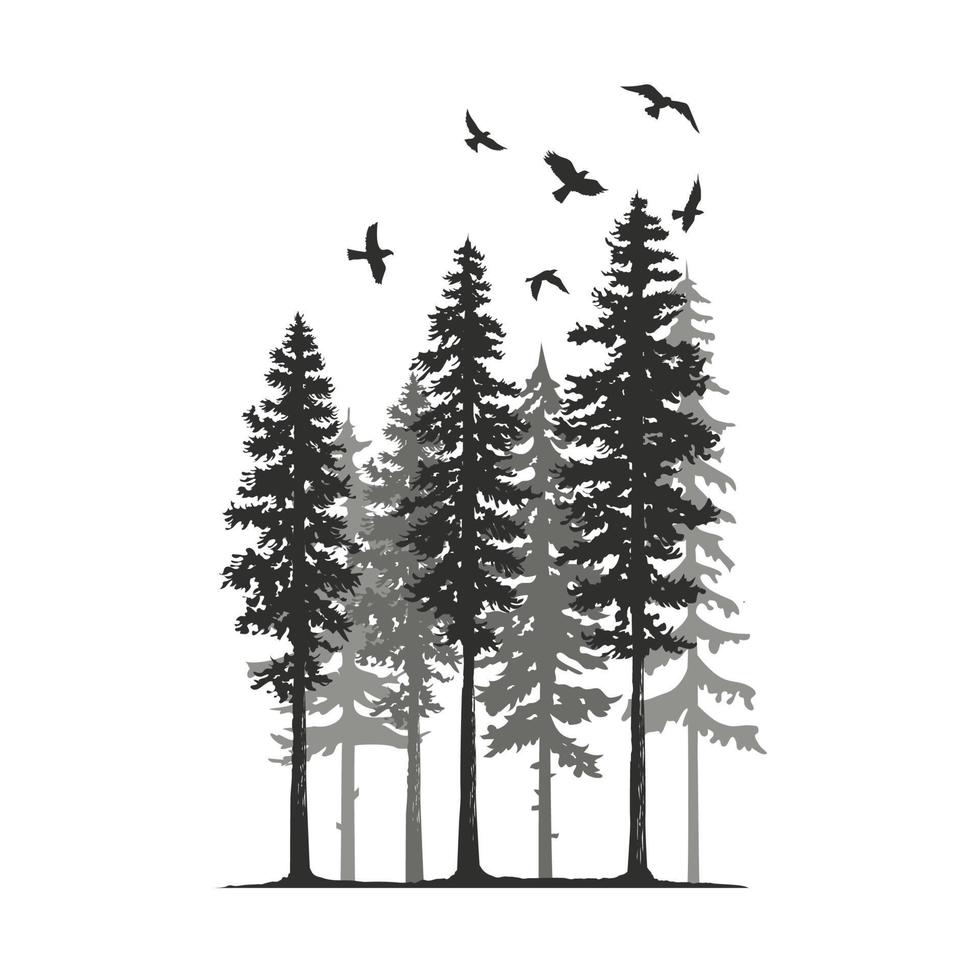This black and white illustration features seven pine trees with varying shades and heights, ranging from very black to light gray. The trees extend from the bottom of the frame to the top, with the lower halves nearly devoid of branches. In the foreground, three of the trees have intensely black trunks and foliage, while the remaining four trees, appearing as though shadowed, are in lighter and darker gray hues. These background trees might be shadows or additional trees drawn behind the main ones. Above this striking forest scene, against a white background, six birds with wings spread, possibly hawks or falcons, fly in silhouette. The composition captures the serene yet dynamic interplay of nature's elements.